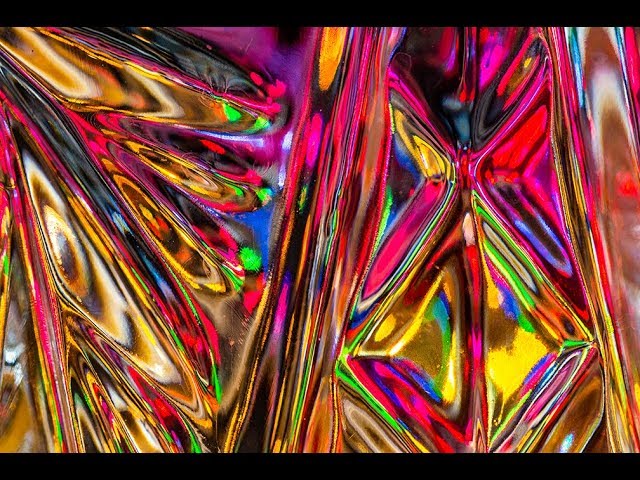The picture is a vibrant and abstract piece, possibly a painting or digital artwork, characterized by a riot of colors including black, gold, yellow, orange, neon green, blue, purple, pink, and red. It has a black stripe running across both the top and bottom borders, framing the chaotic, colorful center. The image appears divided into four sections: two larger ones on the left and two smaller ones on the right.

On the left side, there are elongated, finger-like extensions of paint flowing downwards and slightly to the right, starting with black, purple, and yellow, transitioning into layers of red, green, and more yellow. Further down, these fingers continue with hues of blue, red, black, yellow, and gray.

The sections on the right feature intricate vertical lines and shapes, including a section with vertical lines extending from the bottom upwards, featuring black, yellow, purple, red, and brown. Additionally, there is a notable butterfly-like shape formed by an X pattern, mainly in black and red, with wings displaying purple and yellow on the left, and red, blue, and black on the right, accentuated by red lines and vibrant color streaks.

Further to the right, streaks of yellow, which fade into brown and purple, extend from the bottom at a slight angle. This is contrasted with thicker streaks of brown, white, and blue. The top right corner is minimally adorned with a hint of pink, adding to the kaleidoscopic, somewhat smushed-together appearance that evokes images of peacock feathers or cell clusters, lending the artwork a dynamic and vibrant feel.